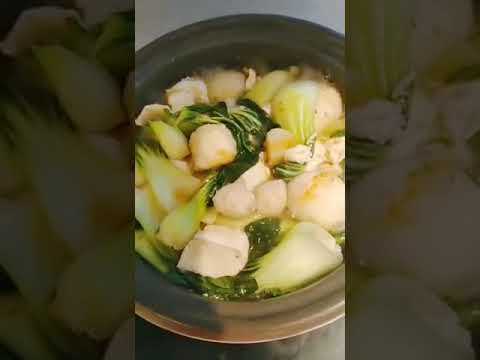The image showcases a detailed culinary scene, prominently featuring a bowl of soup or broth that's brimming with an assortment of vegetables and other ingredients. At the center of the photo is a slightly shiny, silver bowl with a wide lip, filled nearly to the rim. Inside the bowl, large pieces of greens such as spinach, Napa cabbage, or bok choy float in the liquid, alongside white cubes that appear to be tofu. Scattered within the mix are other elements like mushrooms, light green leeks, and possible cubed potatoes, all blending together to form a hearty, vegetarian broth. The bowl rests against a gray, somewhat blurred background, which looks like an enlarged, faded version of the same image, creating a picture within a picture effect. The focal point is the bowl itself, which is positioned directly in the middle of the frame, with no other objects or text present, giving the image a clean, focused look that could easily appear on a social media platform like Tik Tok or Instagram.